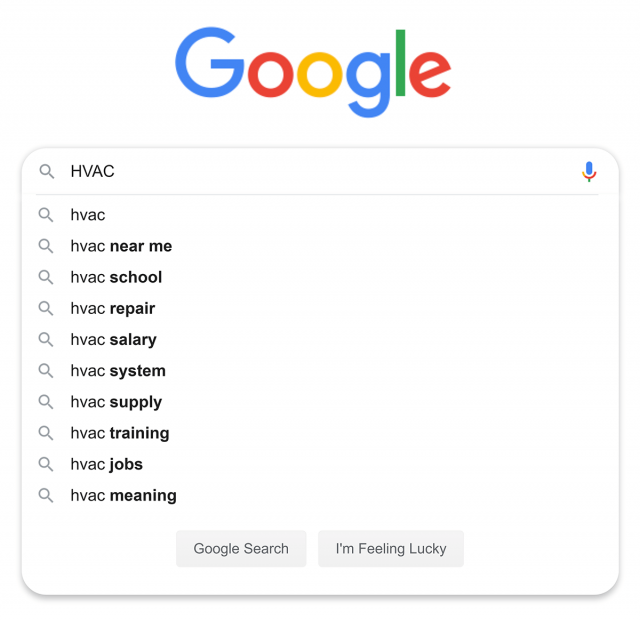The image is a detailed screenshot of the Google search homepage. Dominating the top section of the page is the iconic Google logo, where each letter is rendered in a different vibrant color: the capital G and lowercase g are in blue, the first O and E are in red, the second O is in yellow, and the L is in green. Below the logo, the search bar stretches horizontally across the screen. On the left-hand side of the search bar is a magnifying glass icon, while the right-hand side features a multicolored microphone icon, designed with blue, yellow, red, and green hues that echo the Google logo's colors.

Inside the search bar, the term "HVAC" is typed out in all capital letters. Directly beneath the search bar, Google offers a list of search suggestions. These suggestions begin with "HVAC" in lowercase, followed by related terms such as "HVAC near me," "HVAC school," "HVAC repair," "HVAC salary," "HVAC system," "HVAC supply," "HVAC training," "HVAC jobs," and "HVAC meaning." Each suggestion is accompanied by a small magnifying glass icon to its left.

At the bottom of the screen, there are two rectangular buttons placed side by side. The button on the left is labeled "Google Search," while the button on the right is titled "I'm Feeling Lucky."